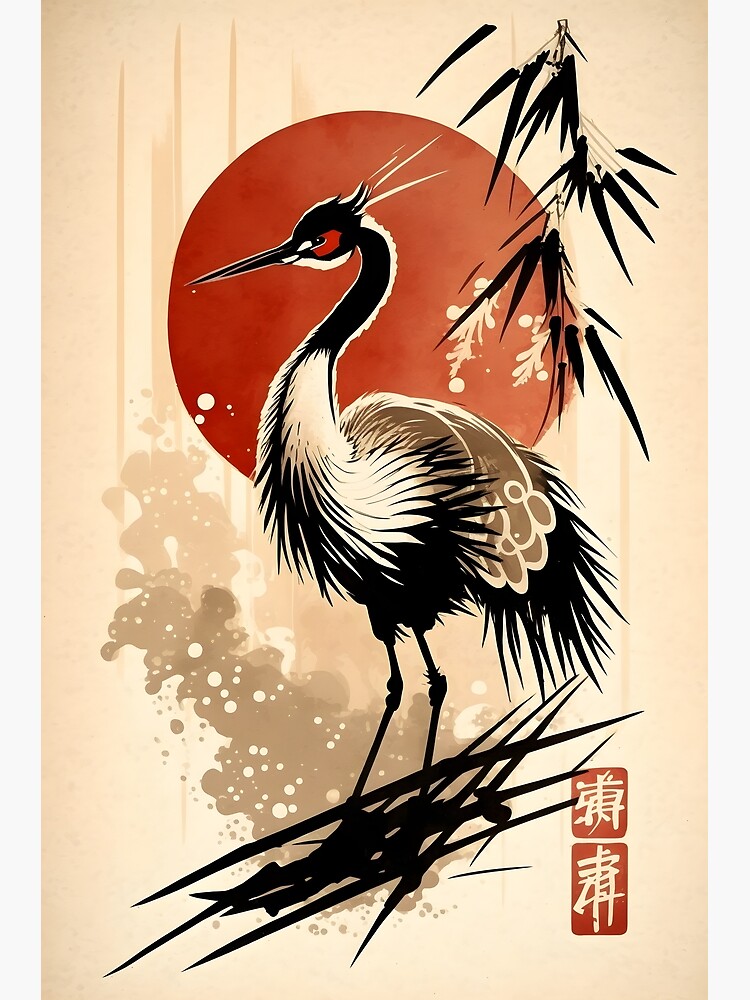This is an Asian-style digital painting depicting a crane in side profile, looking to the left. The crane features a black neck, long black beak, red eye mask, white feathers around its neck, brown feathers towards its back, and a black tail. It stands on two thin black legs amidst a series of intersecting black lines at the bottom of the image, resembling grass. The background showcases a prominent red sun, symbolizing the Japanese flag, with varying shades of red and subtle shadows. Black bamboo leaves cascade from the right side, adding to the Nipponic theme. In the lower right corner, two red boxes contain white Chinese characters, enhancing the artwork's cultural context. The overall color palette is dominated by sepia tones and black outlines, with occasional hints of red.